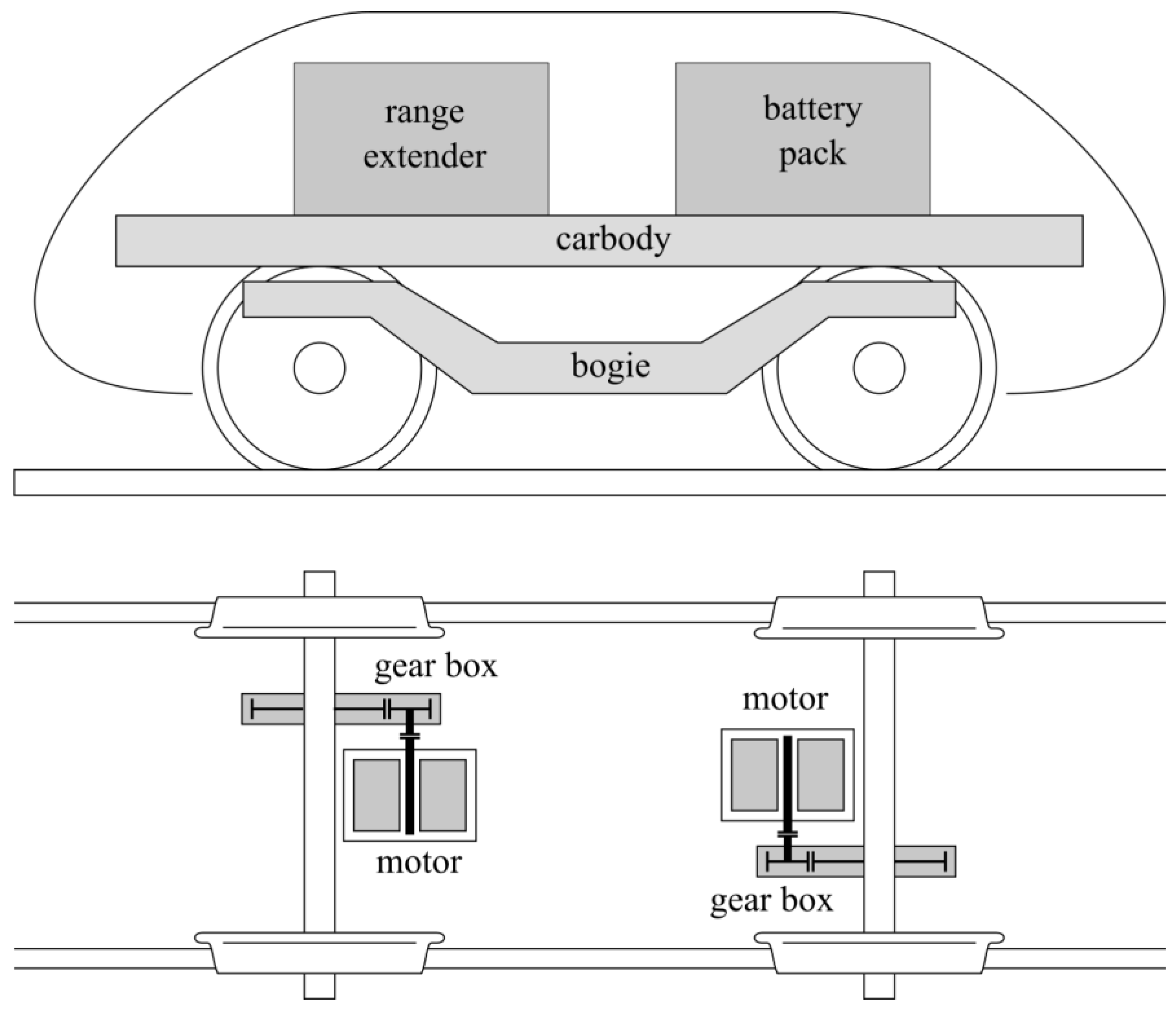The image is a black and white, computer-generated scientific diagram depicting a simplified side view of an electric train car. The diagram features labeled components including a ‘car body’ with a rounded shape, mounted on two wheels connected by a bogie. Positioned on the car body are two boxes; one labeled ‘range extender’ and the other ‘battery pack’. Below this is a depiction of the train car's undercarriage, drawn from a top-down perspective. In this lower portion, two axles on parallel rails are visible, each connected to a gearbox and a motor. The gearboxes and motors are shown as dark gray boxes, with the motors labeled as ‘motor and gearbox’ on the left side and conversely on the right. The sketch utilizes simple line drawings with some gray shading, providing minimal detail.